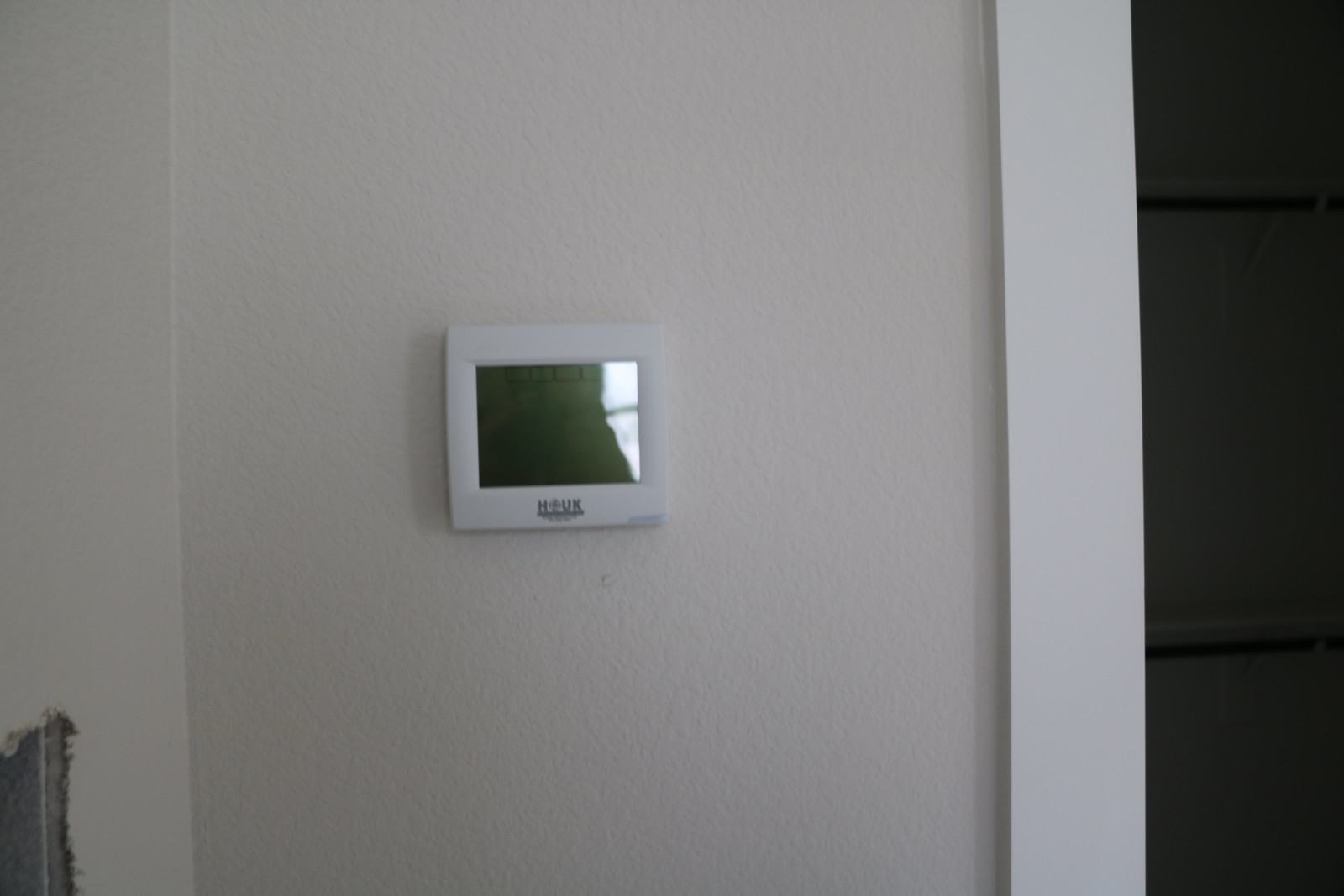The image depicts a section of a room with an off-white textured drywall. The color of the wall appears slightly muted in comparison to the brighter white door jamb adjacent to it. In the bottom left corner of the image, there is a visible hole cut into the drywall, suggesting potential recent work such as accessing wiring or repairing a water leak.

Central to the image is a prominently featured wall thermostat with a noticeably large, square plastic exterior. The brand name on the thermostat, which seems to start with an "H" and possibly followed by a "K," is written in gray lettering and includes a horizontal line beneath it. Above the brand name, the thermostat has a large digital screen displaying information, which appears greenish. However, the screen's details are obscured by a significant glare coming from a nearby window, adding difficulty to viewing the screen's contents. The image quality is slightly grainy, contributing to the overall lack of sharp detail.